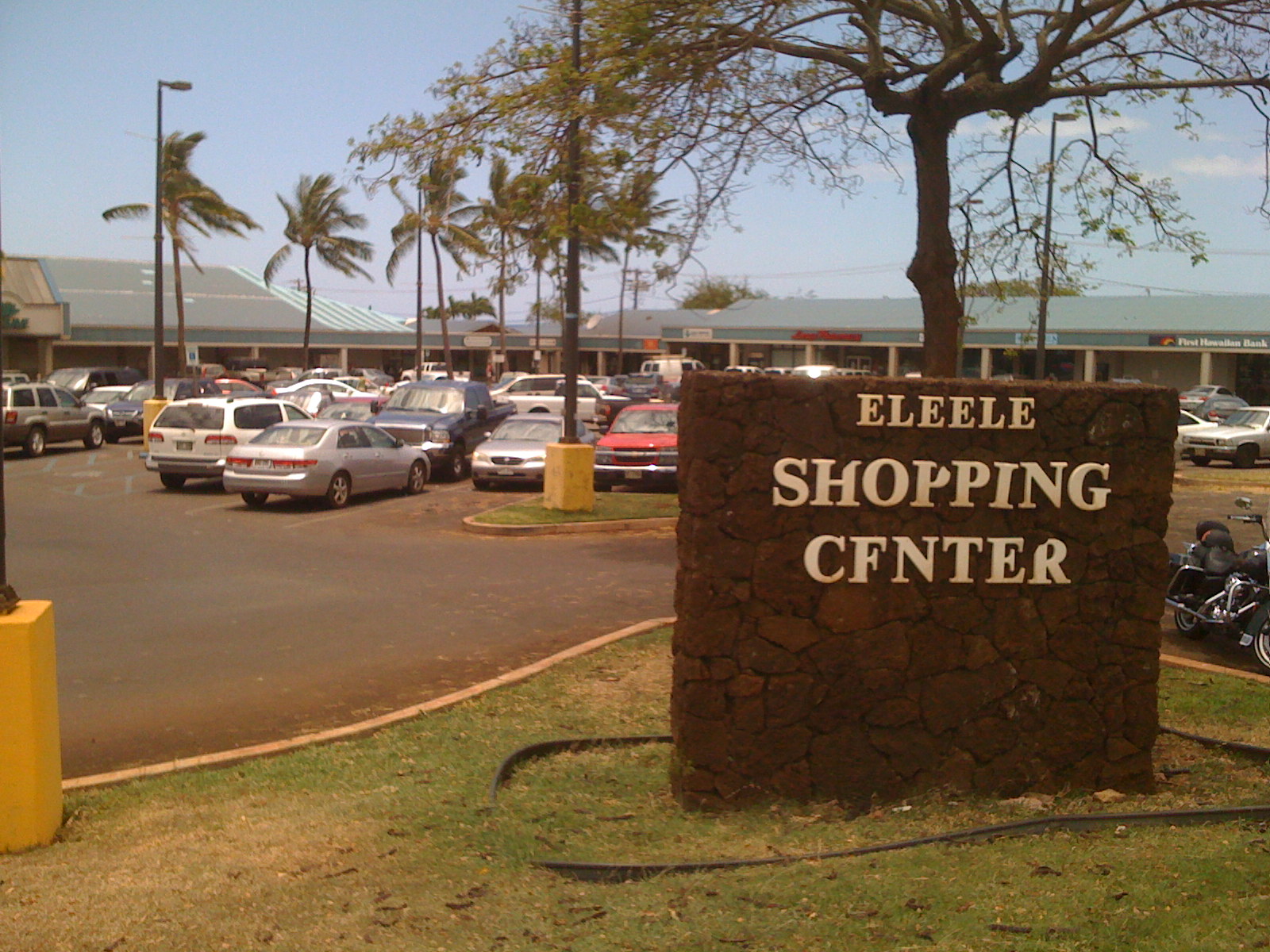This photograph captures a lively scene outside a shopping center, set against a backdrop of a clear blue sky. The single-story shopping center extends from the back left to the back right of the image, featuring a flat, gray roof. A large, nearly full parking lot packed with cars lies in front of the buildings, with several palm trees scattered among the vehicles, adding a touch of greenery to the asphalt. 

In the foreground, slightly right of center, a prominent stone sign made of brown rock stands about three and a half feet tall on a patch of green grass. Although weathered and worn, the sign reads "Ely Shopping Center," though the letters show signs of damage - part of the "H" and "P" in "Shopping" are missing, the "I" in "Center" is tilted, and parts of the "E" and "R" are also worn. To the right of the sign, a motorcycle is parked, adding further detail to this bustling scene.